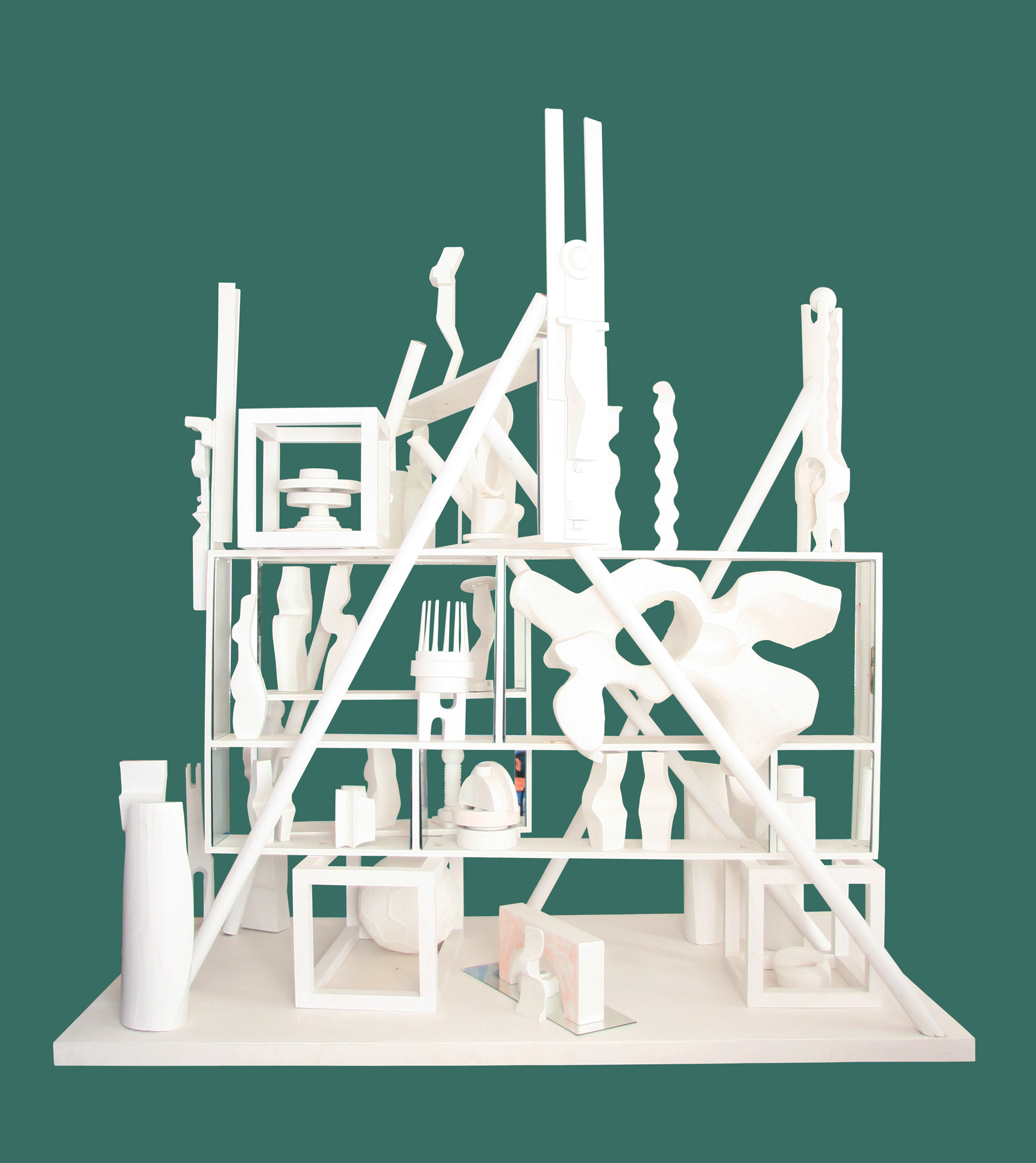The image depicts a vertical rectangular artwork set against a dark greenish-gray background. The centerpiece is an intricate white sculpture resembling a multi-level shelf or structure, crafted from a flexible white material, possibly resembling clay. It is mounted on a flat white base and features several shelves, each populated with a variety of white objects. Noteworthy elements include a tall, round pillar on the front left corner, several diagonal poles, and a vertical squiggly line.

The sculpture houses various abstract shapes and forms across its levels, including spiky objects, cylinders, and rectangles turned on their sides. Notably, the second level features a miniature figurine emerging from a door-like opening, while the topmost level contains images of women and what appears to be a cylindrical tool designed for gripping.

The detailed arrangement captures a sense of an eclectic mix of tools, machine-like parts, and possibly AI-generated elements, contributing an intricate and somewhat surreal aesthetic to the overall piece.